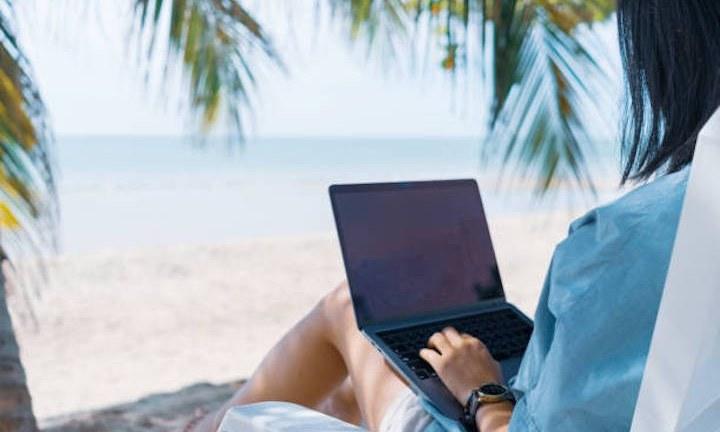In this serene beach scene, a woman is seated facing away from the camera, surrounded by tropical palm trees and overlooking a breathtaking view of the light blue ocean under a clear, sunny sky. She is dressed in a simple sky-blue shirt and white or beige shorts, partially visible from just above the ankle. The woman is sitting comfortably in what seems to be a white vinyl beach chair with her feet in the sand. Her left hand, adorned with a watch, rests on the keys of an open laptop on her lap, although the screen remains dark. The faint and hazy horizon adds to the tranquil atmosphere, as the green palm fronds gently hang around her. In the bottom of the frame, there's a tiny glimpse of sand, further enhancing the overall peaceful and relaxing setting.